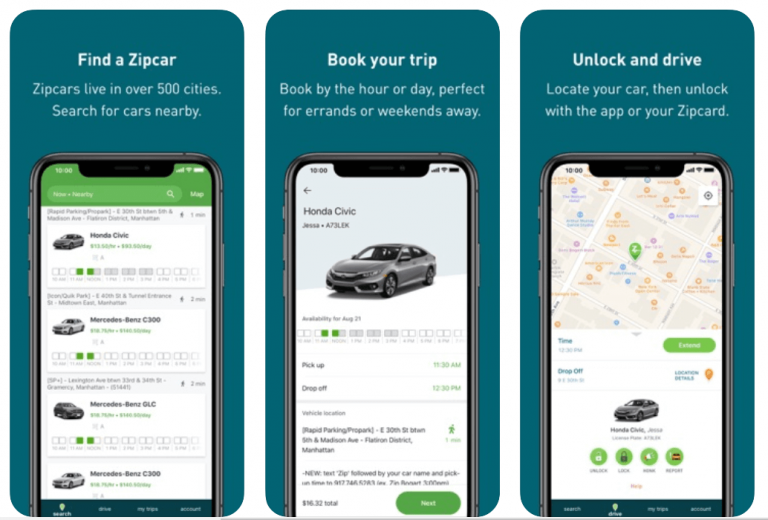The image showcases a modern app or website interface designed for car rentals, likely for the popular service Zipcar. The top section features a search function captioned "Find a Zipcar," highlighting that Zipcar operates in over 500 cities. The middle of the image shows a smartphone displaying various available car models, including a Honda Civic, Mercedes-Benz C300, and Mercedes-Benz GLC. Captions such as "book your trip" indicate that users can rent cars by the hour or day, ideal for quick errands or longer weekend getaways. Below, another smartphone image illustrates the booking process with a clear depiction of a Honda Civic, emphasizing the "pick up" and "drop off" steps. The final section explains the convenience of unlocking the rental vehicle via the app or a Zipcard, with a map interface on the phone displaying the car's location, labeled possibly with "expand" in a green box.